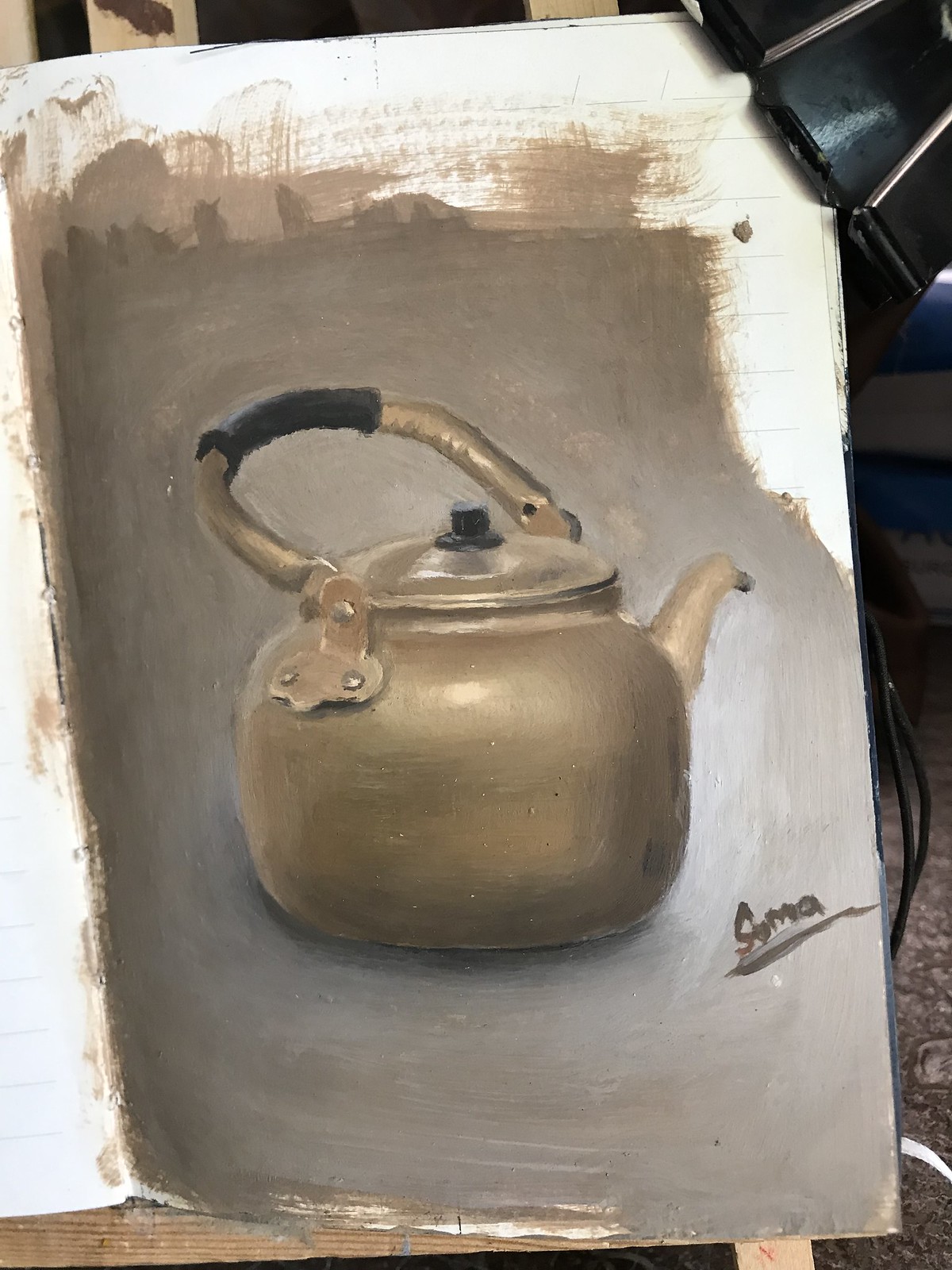A meticulously rendered oil painting on a clean white canvas showcases a still life scene featuring a vintage bronze kettle. The kettle is adorned with a lid, topped by a small black knob, and possesses a functional handle encased in a black rubber grip for ease of use. The spout is strategically positioned facing away from the viewer, adding a touch of intrigue to the composition. The artist, whose signature "Soma" is elegantly inscribed in brown at the lower right corner of the canvas, has chosen a backdrop of muted brownish-gray tones, lending the scene a timeless and contemplative atmosphere.